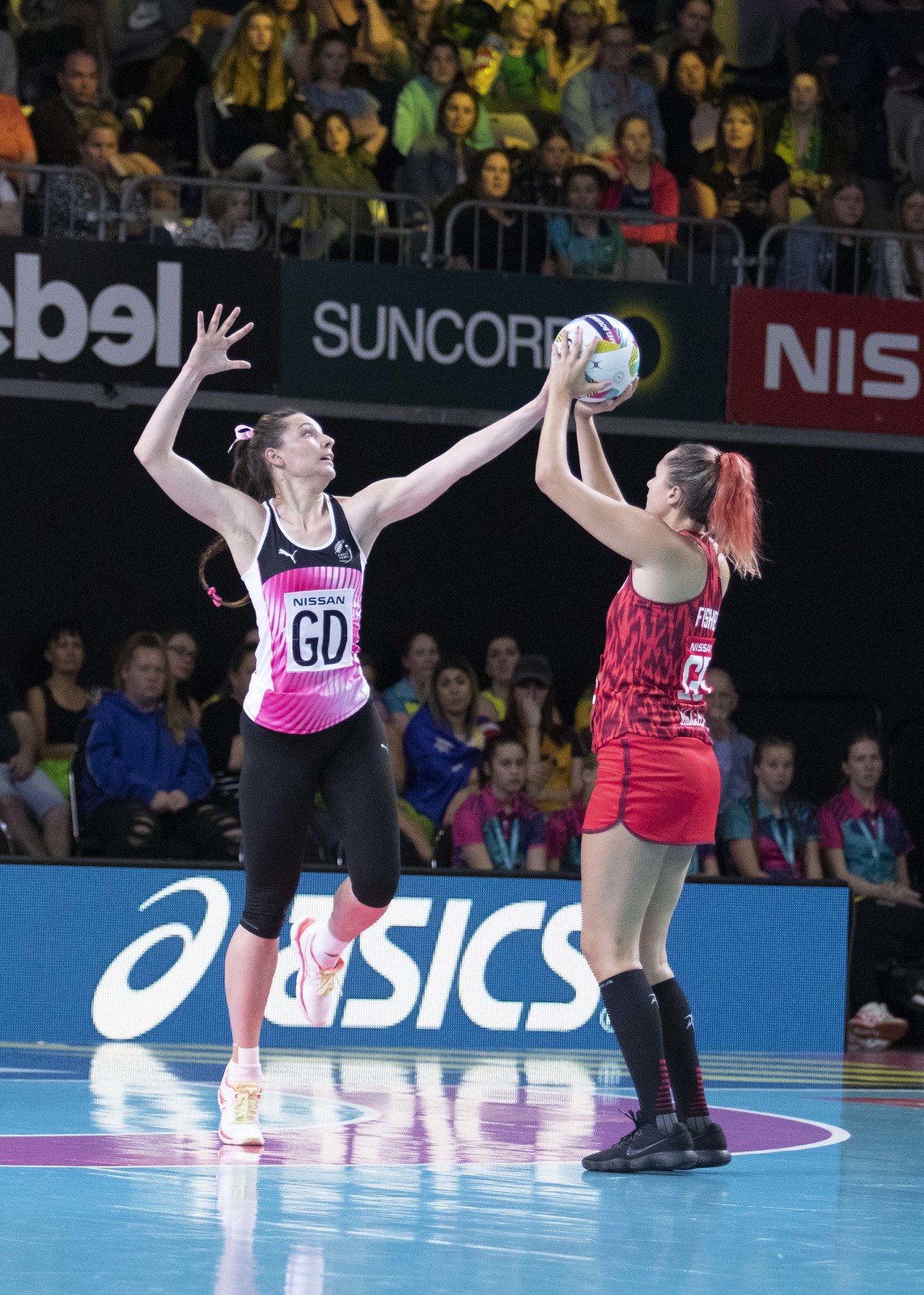The image depicts a vibrant scene on a volleyball court, repurposed from a basketball rink and surrounded by an enthusiastic audience. In the foreground, two young women in their 20s are the central focus, seemingly demonstrating volleyball skills. The court features colors of blue and purple and is prominently sponsored by ASICS, with a large banner displaying the brand. 

One woman, positioned on the right side, is dressed in a pink and black tank top paired with black capris. She has one arm raised, poised as if to serve or spike the ball, her other arm pulled back, and one foot slightly lifted off the ground. Her counterpart on the left is in an all-red uniform consisting of a red tank top, red shorts, black knee socks, and black shoes. She is holding the volleyball with both hands, possibly preparing to serve. 

Partial signs with names like Suncor and Nissan are visible amidst the crowded stands, indicating a large event or tournament setting. Despite the lack of a visible net, the scene vividly captures the energy of a volleyball match or a skill demonstration, with the players showing intense focus and readiness.